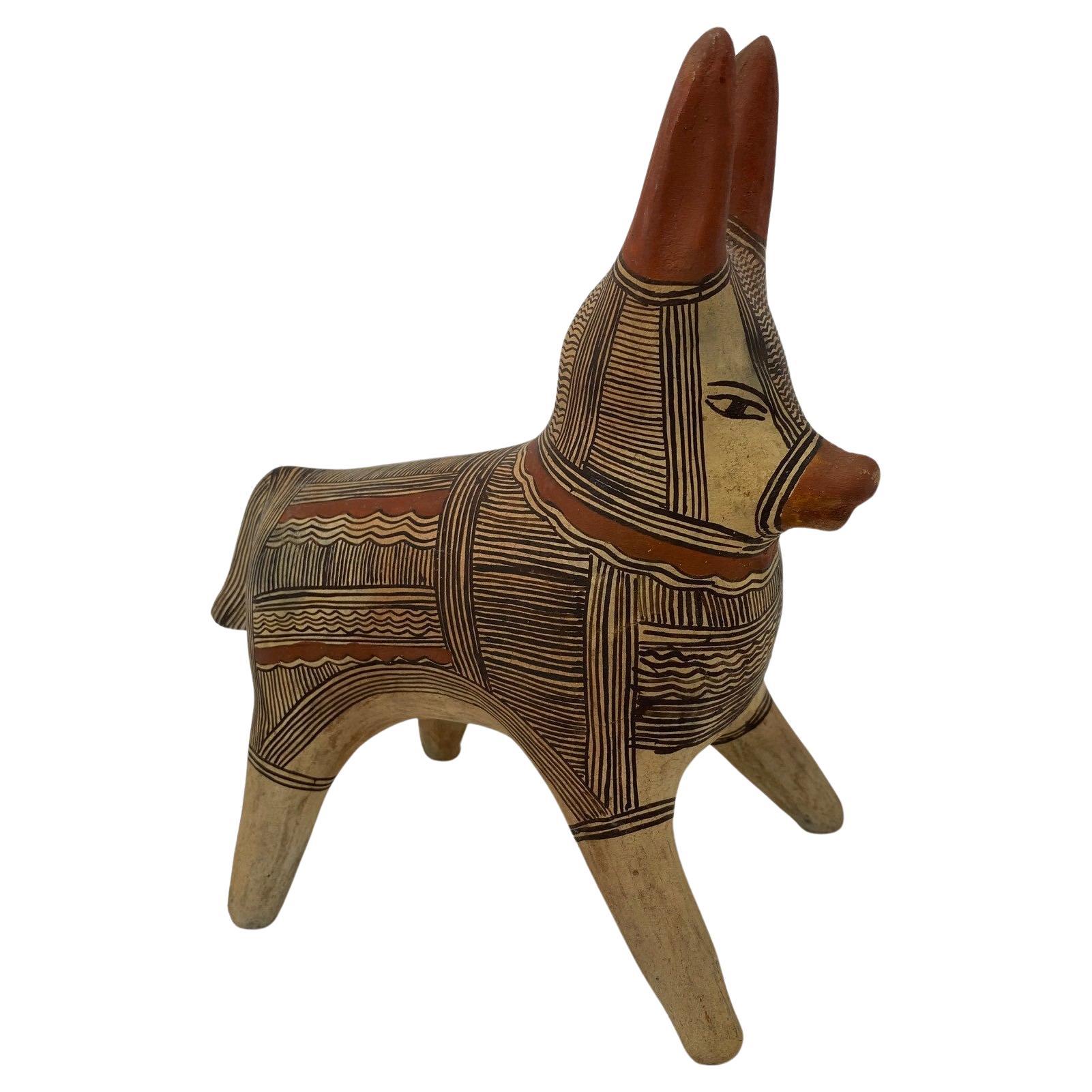This vertical image captures a meticulously carved wooden statue of a dog. The statue features very large, upright ears that almost reach the length of its legs, both of which are smoothly finished in a burnt sienna color at the bottom. The dog's body is intricately adorned with horizontal black lines and vertical strap-like circles in opposing directions, creating a complex pattern across the wooden surface. Adding to the vivid detailing, the dog has red elements: its snout, ears, a ring around its neck, and several stripes on its back. The face of the dog appears to have a hood-like structure over its ears, with an eye painted on it, contributing to the sense that it is more of an artistic toy or material-made figure than a realistic animal. The tail, although partially turned towards us, continues the theme of detailed carving, complementing the overall aesthetic of the statue.